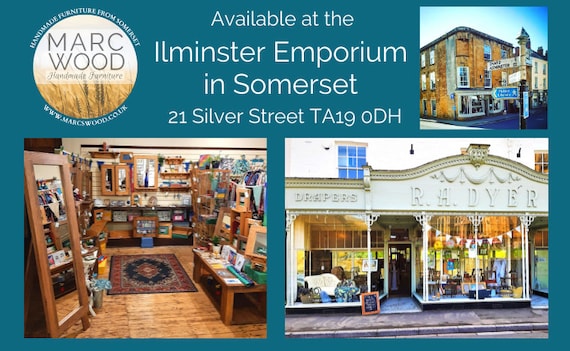The image is a detailed advertisement for Mark Wood Handmade Furniture, available at the Ilminster Emporium in Somerset, located at 21 Silver Street, TA19 ODH. The ad is rectangular, measuring approximately four inches wide by three inches high. The background is a greenish-blue color.

In the upper left corner, there is a circular logo. The lower half of the circle features golden wheatgrass, while the upper half is white, displaying the text "Mark Wood Handmade Furniture" in gray. Above the circle, the text "Handmade Furniture from Somerset" is printed in blue. Below the logo, the website "www.marcswood.co.uk" is provided.

Prominently in the center, the text in large blue print announces the availability of the handmade furniture at the Ilminster Emporium in Somerset, including the detailed address.

In the upper right corner, there is a square photograph of a brick building with street signs in front of it. Below this, there are two additional photographs. The left photo captures the interior of the store, showcasing various items for sale, including a beautifully crafted wood interior. The right photo portrays the exterior of the store, a white-fronted building bearing the sign "Drapers are a Dyer."

This advertisement effectively combines detailed text and images to promote Mark Wood Handmade Furniture at the Ilminster Emporium.